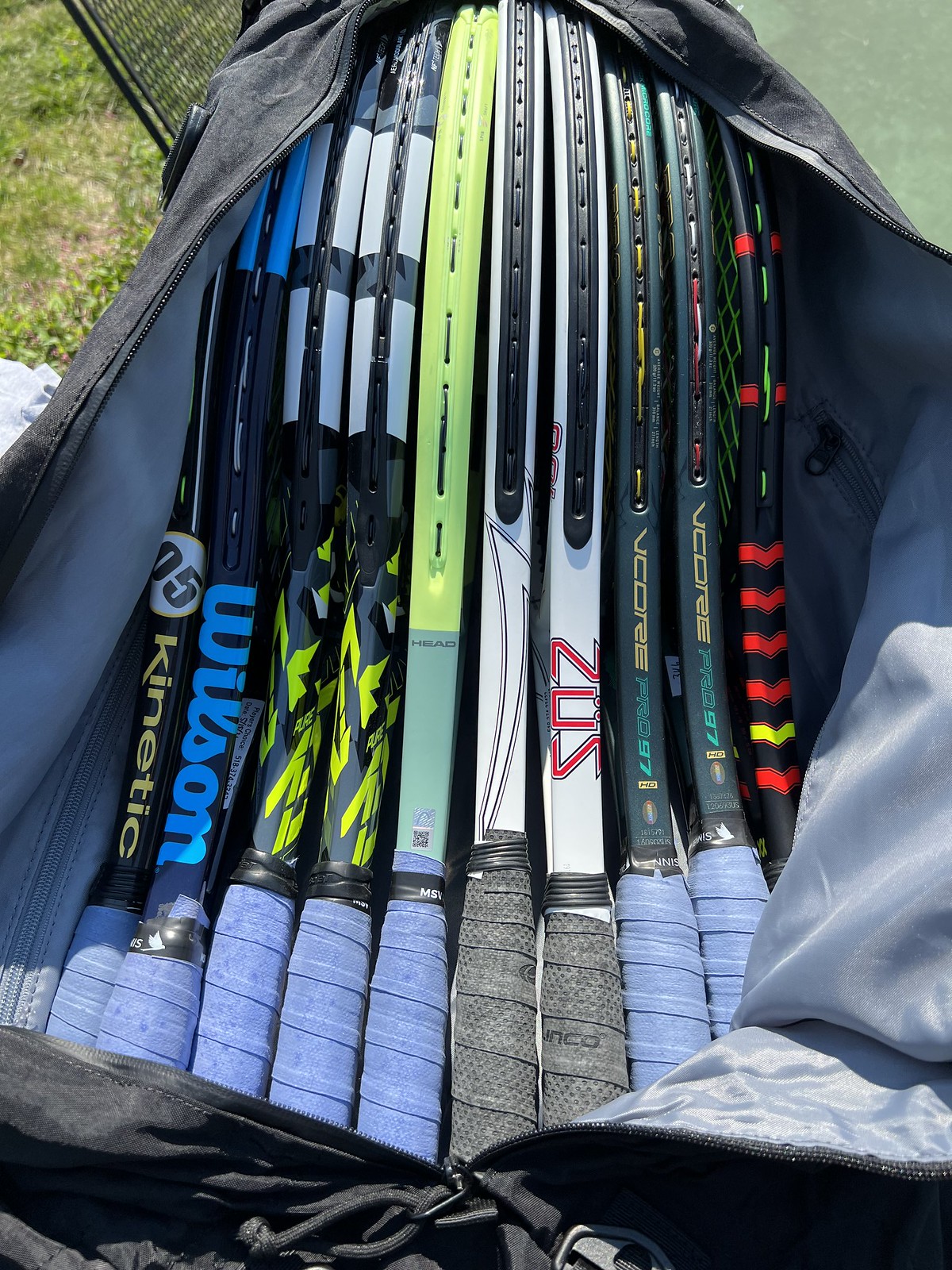The image is a well-lit outdoor scene featuring an open black duffel bag containing a variety of tennis rackets. The bag is unzipped and lies on a flat surface, with grass visible in the upper left corner, indicating it’s taken outside on a sunny day. Inside the bag, there are 10 tennis rackets neatly stacked on their sides, allowing for their brand names and designs to be visible. Most of the racket handles are wrapped in blue tape, except for two in the center which have gray tape. The rackets are primarily black with other colors and designs, including brands like Wilson, Kinetic, Zoss, and V-Core. One notable racket on the right side has red and yellow arrows on it, while others have various color schemes such as black and lime green, white, and black with blue lining. The bag itself is black with a gray interior, and its sides are folded out, revealing the entire collection of rackets inside.